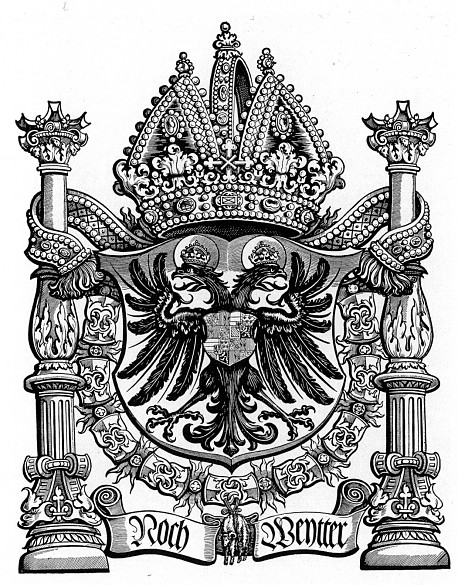This is a highly detailed, black and white pencil sketch depicting an ornate coat of arms. The image is symmetrical, featuring intricate designs and elaborate elements on both sides. Flanking the central figure are two identical columns, each round at the bottom with ornate, three-pronged tops. These columns have classic marble-like fluted lines running vertically. Interconnecting these columns is a bedazzled, tasseled ribbon that enhances the regal appearance of the image. 

Central to the coat of arms is a shield, behind which stands a majestic, two-headed phoenix-like bird. Each head faces opposite directions – one to the left and one to the right – and both are adorned with small crowns. The bird's large wings are spread wide, and its claws are extended, showcasing sharp talons. Above this central figure sits a three-pointed jeweled crown, further embellished with small circles mimicking jewels.

At the bottom of the illustration, a filigreed scroll contains the text "Roche-Benter," inscribed elegantly. This elaborate design combines traditional heraldic elements with luxurious details, making it an impressive and visually captivating coat of arms.